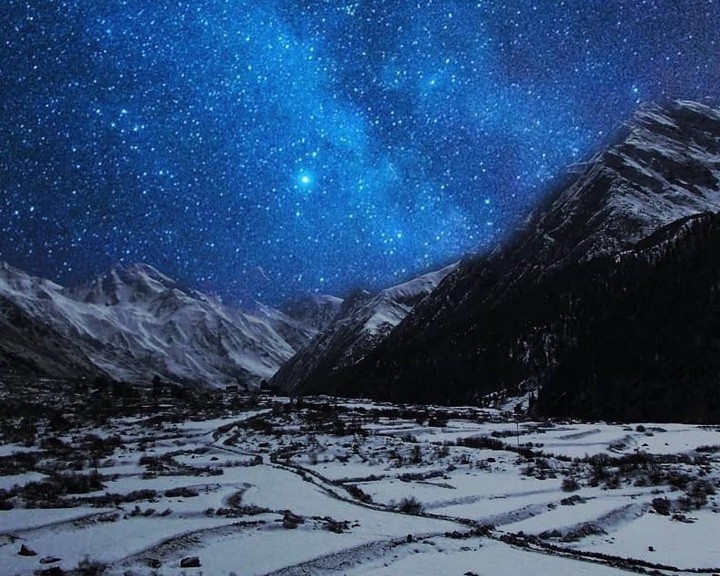The image depicts a stunning computer-generated painting of a snow-covered mountainscape at night. Dominating the background, the rocky, tall mountains are capped with snow and set against a deep blue-black sky, sparkling with countless stars and a prominent north star. Below the majestic mountain range lies a serene, flat valley or plains, blanketed in snow. This valley features a small village or city with scattered houses, interconnected by little roadways and nestled amid snow-covered ground. A river winds diagonally through this snowy landscape from the bottom right corner, adding a natural flow to the peaceful scene. Tall, snow-dusted trees are dotted throughout the village and alongside a main road that cuts through the valley, leading in and out of the scene, enhancing the secluded, tranquil ambiance of this picturesque winter night.